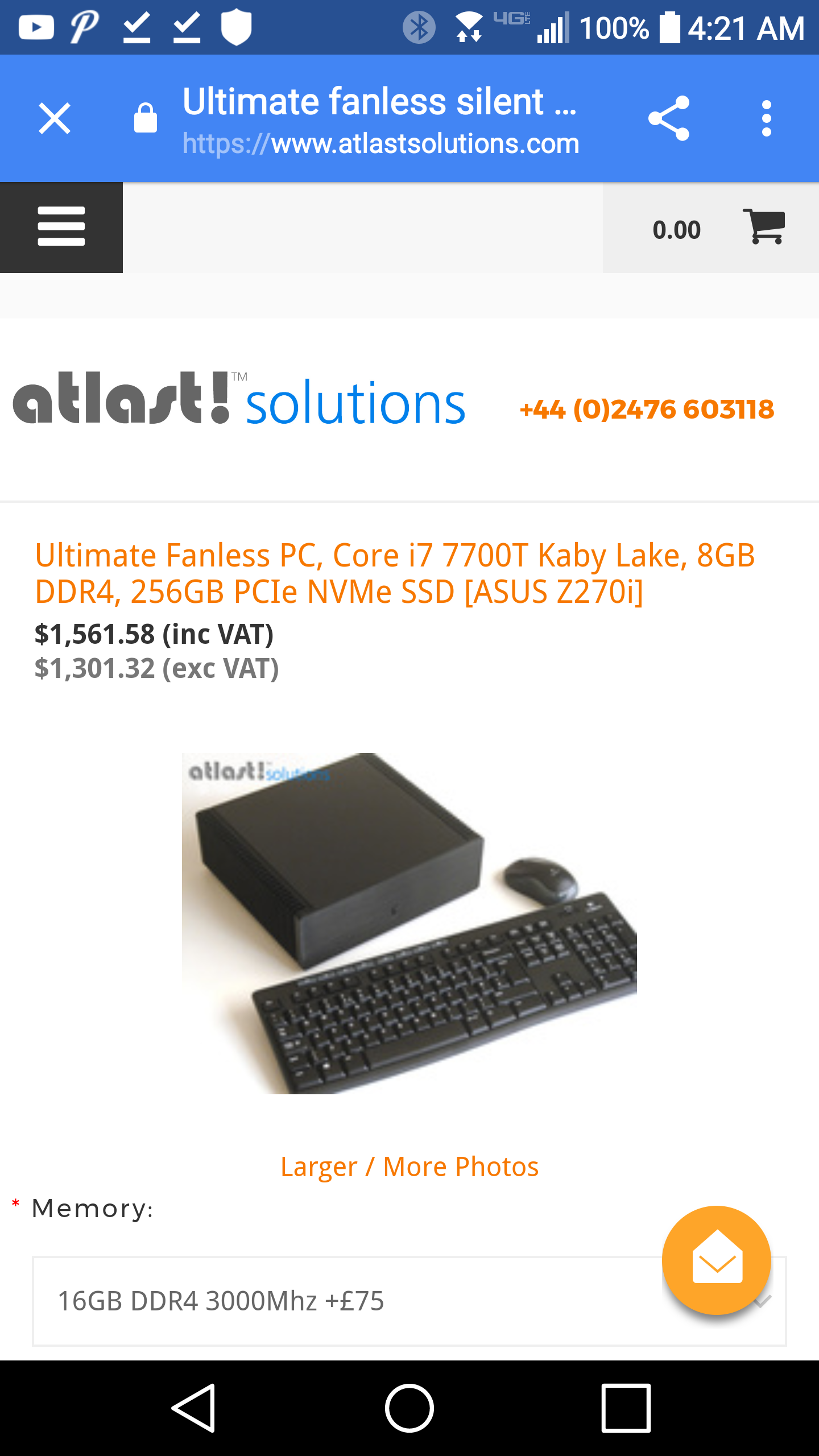This is a screenshot of a web page viewed on a cell phone. At the top of the page, there's a blue rectangular horizontal bar. On the left side of the bar, there's a white 'X' icon, followed by a white lock icon. Moving further to the right, it reads "ultimate fanless silent," with three dots following the text. Below this, the URL "https://www.atlas-solutions.com" is displayed. To the far right of the blue bar, there is a white share icon and three vertical dots.

Below the blue bar, the text "Atlas Solutions" is prominently displayed, with "Atlas" in dark brown, an exclamation mark, and "Solutions" in blue. To the right of this, there is a phone number: 440-247-660-3118.

The main content of the page includes the title in orange text: "Ultimate Fanless PC Core i7-7700T Kaby Lake 8GB". Beneath this, detailed specifications are listed: "DDR4, 256GB PCIe NVMe SSD, and Asus Z270i". Further down, the price is noted as "$1561.58 INC VAT". Below this, "EXC VAT" is listed as "$1301.32".

An image towards the bottom of the page appears to show a black mouse, a black keyboard, and a desktop computer.